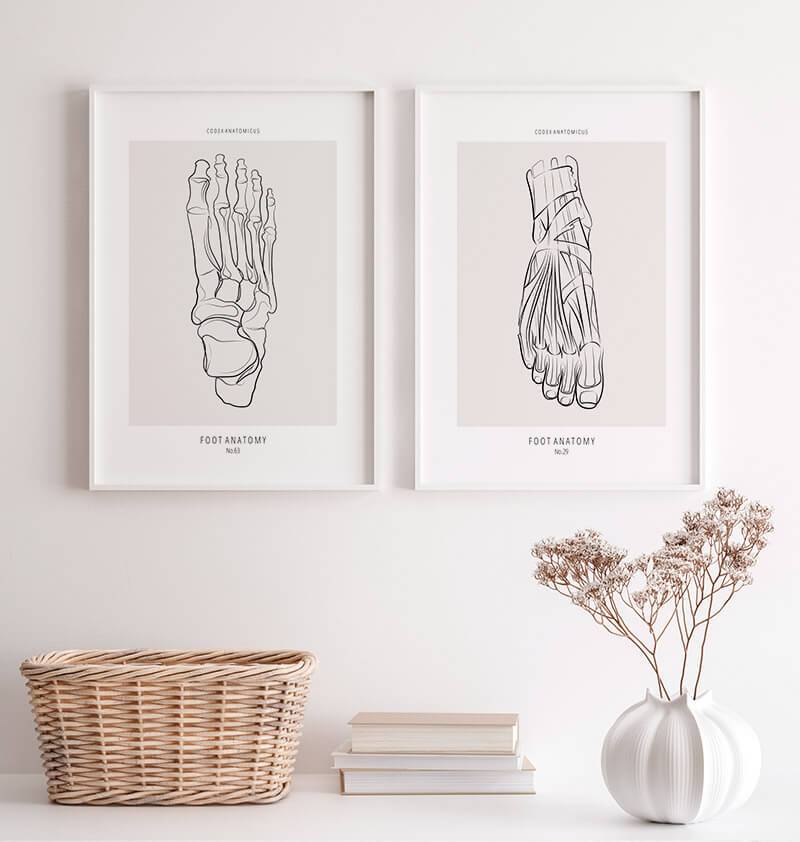This photo captures a modern, white-themed office that might be a doctor's office or belongs to someone with an interest in anatomy. The background features a pristine white wall decorated with two artistic sketches of human feet, both titled "Foot Anatomy." The left sketch displays a skeletal foot with long toes, facing upward, while the right one depicts a muscular foot facing downward, complete with skin and nail details. Below these sketches, a white shelf houses a few items: on the left is a beige rectangular wicker basket, in the middle are three small, old-timey looking books stacked with their pages showing, and on the right is a silvery-white vase resembling a pumpkin, holding a cherry blossom-like plant with white flowers and brown stems. The overall aesthetic is clean, detailed, and somewhat clinical.